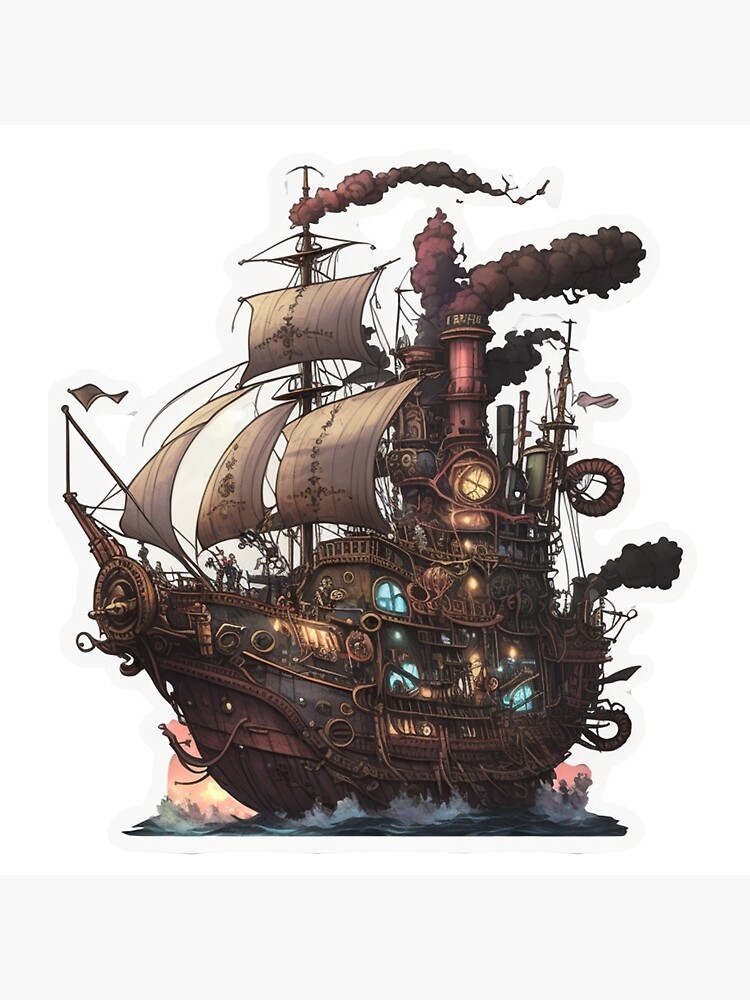The image is a detailed and colorful illustration in a rectangular format, measuring about six inches high and four inches wide, with light gray borders at the top and bottom. At its center is a steampunk-style sailing ship, slightly askew with the left bow closer to the viewer. The ship, constructed of wood and metal in mostly dark hues, sails through dark blue waters with white waves splashing at its sides. It features four sails: two rectangular and two triangular, adorned with indecipherable symbols. These beige-colored sails are attached to a large vertical mast. The ship also boasts steam engines in the center with black smoke billowing out, indicating a fantastical, almost magical energy within. Blue porthole windows dot the vessel, adding to its otherworldly appearance. The illustration appears to be part of a fantasy or game world, emphasizing its steampunk aesthetic with intricate, unrealistic details such as a bronze-colored wheel-shaped crank and an overall design suggesting it is more fantasy than a feasible nautical craft.